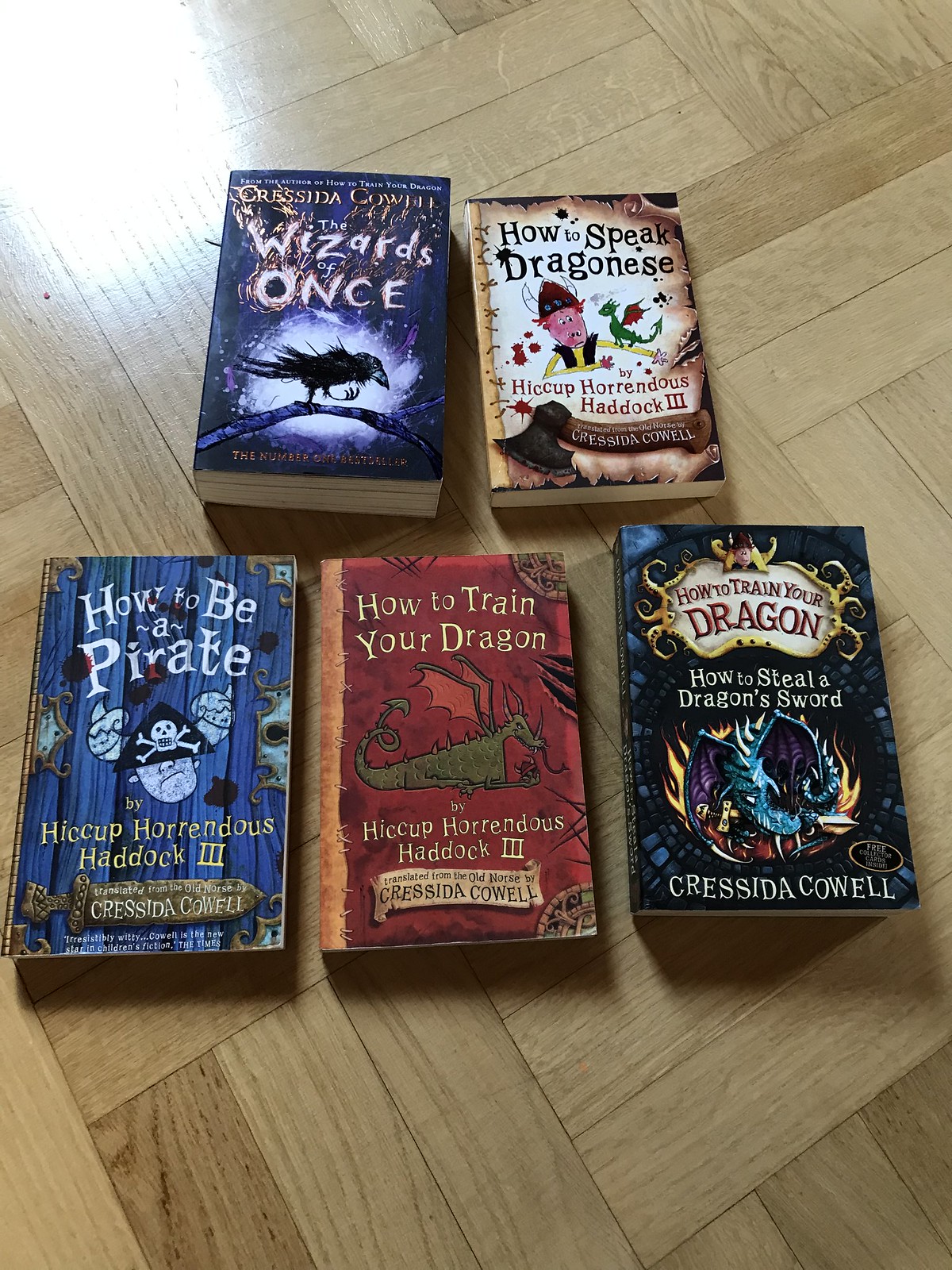Five books by Christina Cowell are carefully arranged on a light parquet floor, illuminated by a bright reflection in the top left corner. On top are "The Wizards of Once," featuring a raven perched on a branch against a circular blue and black background, and "How to Speak Dragonese," showcasing a cartoony boy with a dragon on his arm. Below them, from left to right, are "How to Be a Pirate," depicting a pirate with a captain's tricorne, "How to Train Your Dragon," highlighted by a red cover with a green dragon, and another "How to Train Your Dragon" with a blue dragon and fiery background. The books, distinct in cover art yet unified by fantasy-themed illustrations, display varying hues and fantastical creatures.